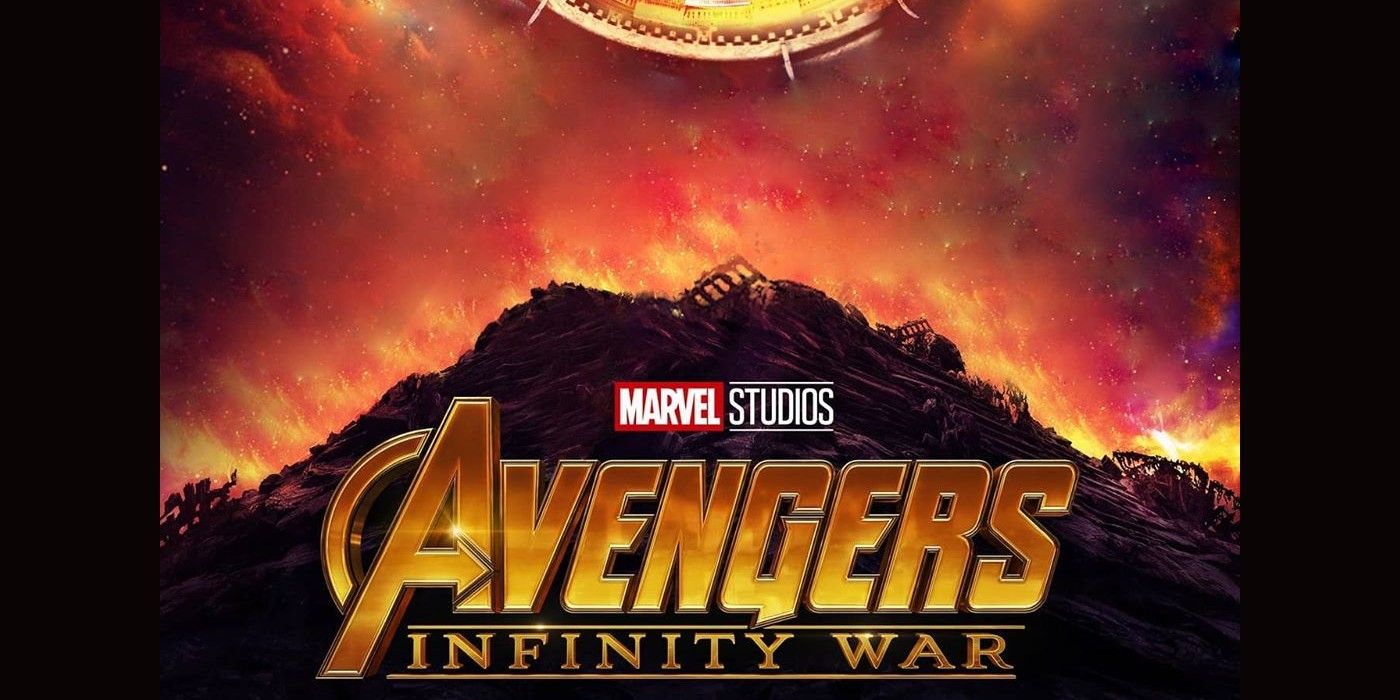This image is a striking, full-color movie poster for Marvel Studios' Avengers: Infinity War. The poster prominently features the Marvel Studios logo mid-image, with 'Marvel' in bold, capitalized white letters on a red background to the left, and 'Studios' in a thinner, capitalized white font on a black background, flanked by horizontal lines above and below. Centered below this, the movie title 'Avengers' is rendered in large, 3D golden letters with a gradient effect, the crossbar of the 'A' styled as an arrow pointing to the right, enhanced by a subtle arch on the left side. 'Infinity War' appears beneath in smaller, 3D golden letters, also featuring underlining. 

The background adds an intense atmosphere with a turbulent sky filled with swirling red smoke, vivid flames, and cinders, suggesting a scene of destruction and mayhem. A mound of debris, possibly remnants of a destroyed structure, sits beneath the tumultuous sky, further adding to the chaotic setting. The overall image has high clarity and ample lighting, giving it a fierce and dramatic feel. No other texts or numbers are present, and vertical black borders frame the left and right edges of the image.